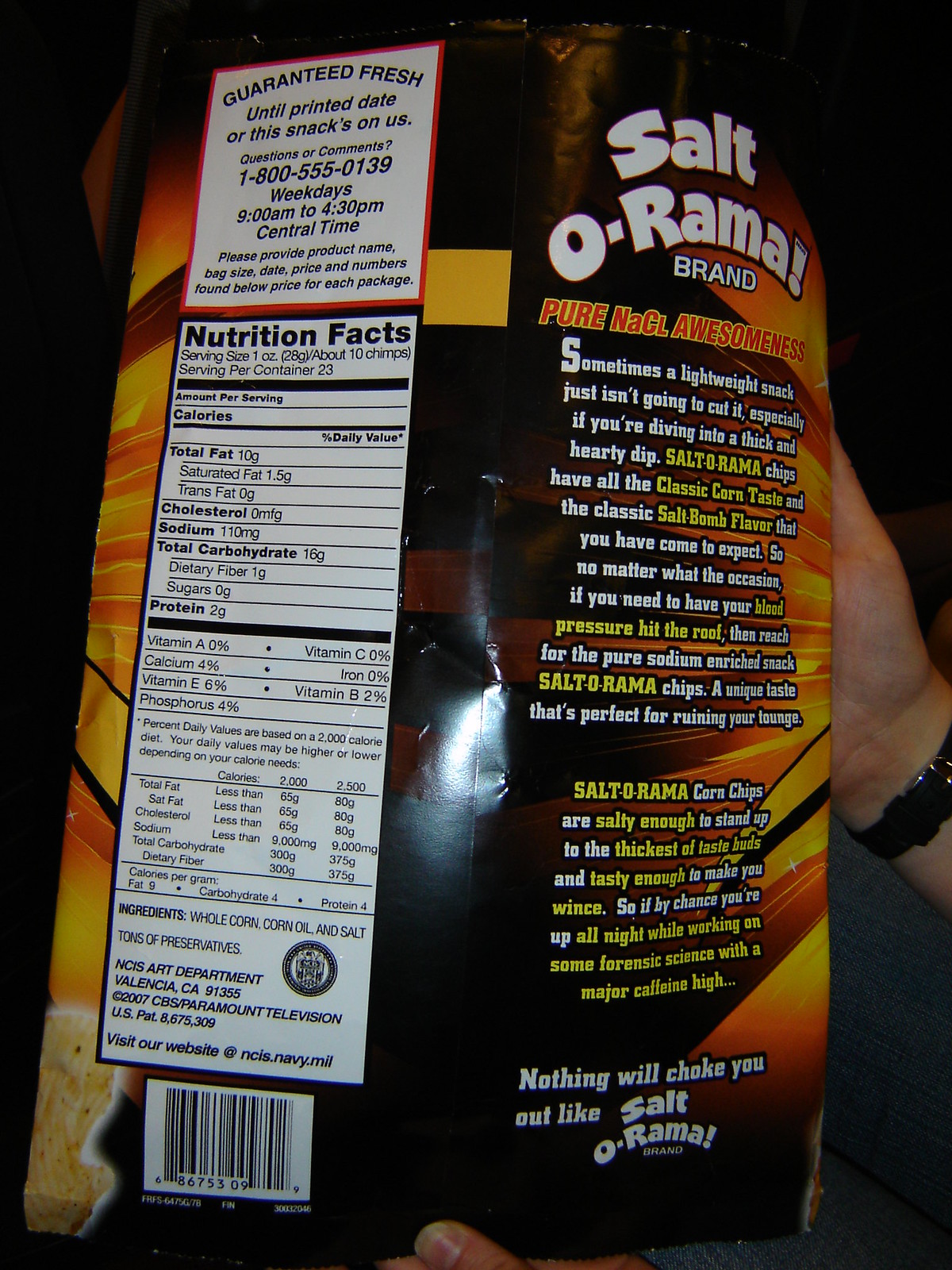The image captures the back of a Salt-O-Rama brand chip bag, labeled as "Pure Knuckle Awesomeness." This indulgent snack boasts a unique flavor profile, perfectly combining the classic corn taste with an intense salt bomb flavor. The bag suggests that whether you're craving a lightweight snack or something more substantial, Salt-O-Rama chips promise to deliver. Described humorously as the snack to reach for if you're aiming to spike your blood pressure, these chips provide a sodium-rich experience that's sure to leave a lasting impression on your taste buds.

Salt-O-Rama corn chips are designed to satisfy even the most robust of taste buds, offering a tongue-tingling experience that might make you wince. The playful description implies that these chips could keep you alert during an all-night forensic science session, complementing a caffeine high to help you power through your work.

The nutritional information indicates each serving contains 10 grams of fat and a substantial 110 grams of sodium, though the calorie count is not specified. Vitamins and other nutrients are minimal.

Visually, the bag features a dramatic design with a dark background accented by streaks of yellow, red, and orange, creating a flame-like impression. The bag is held by a human hand with white skin and a black watch worn on the wrist. The background of the image is black, highlighting the reflective light that draws attention to the center of the chip bag.